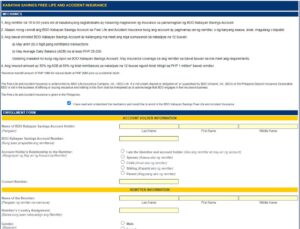This image appears to be a highly condensed and unreadable screenshot of a web-based form. Dominated by a blue and yellow color scheme, the layout features a prominent blue bar at the top with yellow text, followed by a narrower blue bar with white text. Below these headings, there is a white section containing three bullet points and a partial paragraph. Another blue bar with white text is situated further down the page. Underneath the initial yellow bar is a form, likely requiring user input, which includes empty text boxes and checkboxes. A subsequent yellow bar divides the form into additional segments, presumably for more input fields. The overall compactness of the image renders its content largely illegible, with attempts at enlargement resulting in excessive blurriness. The visual story conveyed is one of a structured, yet densely packed web form, marked by its distinct color coordination and multiple interactive elements.